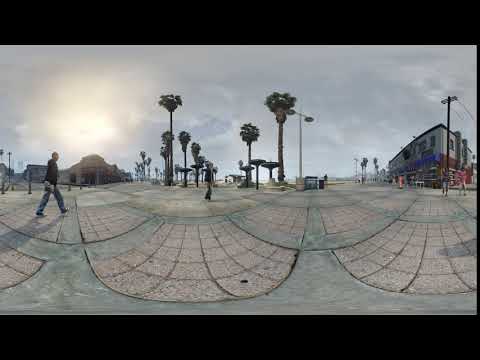The image is a smaller, horizontally-aligned rectangular photo with thick black borders at the top and bottom. The upper part of the picture depicts an overcast sky blending gray and white clouds, with the sun faintly visible behind the white clouds in the upper left corner, creating a somber, rainy atmosphere. Below this sky is an outdoor paved area, a possible town square or park, featuring a mix of light gray pavement and light red bricks arranged in a pattern. 

Centered in the image are several tall palm trees and lampposts. On the left side, a person in a dark top and blue jeans walks towards the right, holding an indistinct object. In the background, the left side of the photo reveals a building situated further away, while the right side showcases a tall building with a gray facade and black roof above a brown base, accompanied by a utility pole and a light gray garbage can in front. Additional power lines and more pedestrians can be seen walking on the right. The scene conveys a sense of dreariness under the heavy clouds, further accentuated by the hint of sunlight struggling to break through.